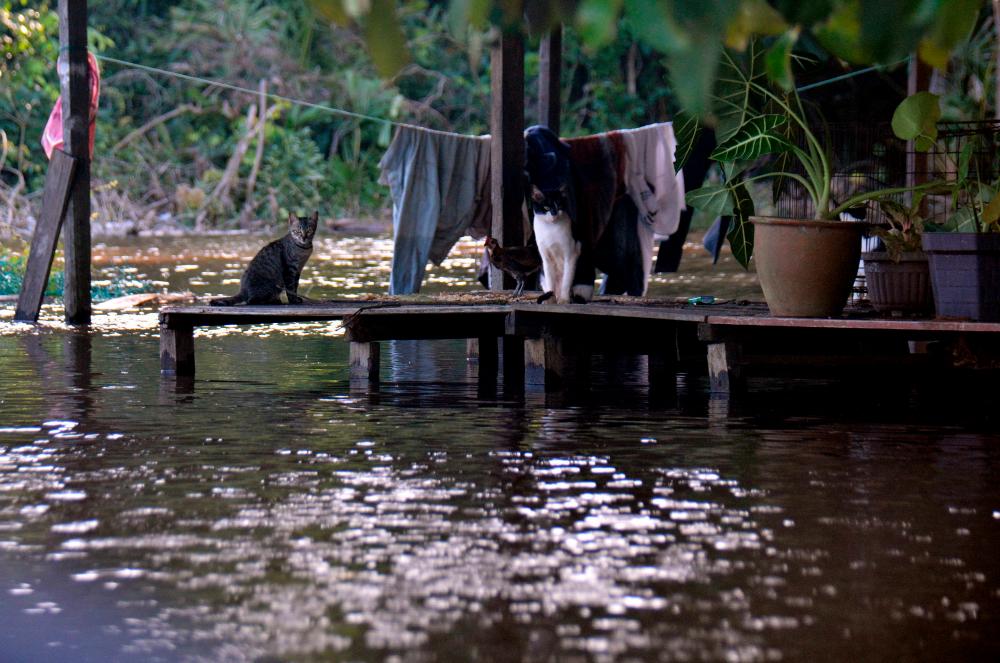The image depicts a rustic, possibly flooded wooden dock or porch, partially submerged in brownish water, suggesting a village setting. Dominating the scene is the water, which surrounds the structure and gives the impression of a gentle, non-rapid flow. The dock, constructed from planked wood on wooden posts, appears weathered and is accompanied by benches, hinting at prior use before any flooding. In the background, a shore lined with thick woods and dense vegetation is visible.

Hanging behind the dock is a clothesline adorned with various linens in shades of gray, white, and brown. Potted plants with lush greenery are situated on the right, adding a touch of vibrant life to the setting. On the dock, an assortment of animals adds a bustling yet serene atmosphere; a lone cat is positioned to the left, while another black and white cat stands alert with a chicken nearby. Additionally, a dog is present, giving the impression of a harmonious coexistence among the animals. The cats are notably attentive, staring directly at the camera, creating a captivating focal point. The combined elements of water, vegetation, and domesticated animals suggest a tranquil yet resilient rural life touched by the encroachment of water.